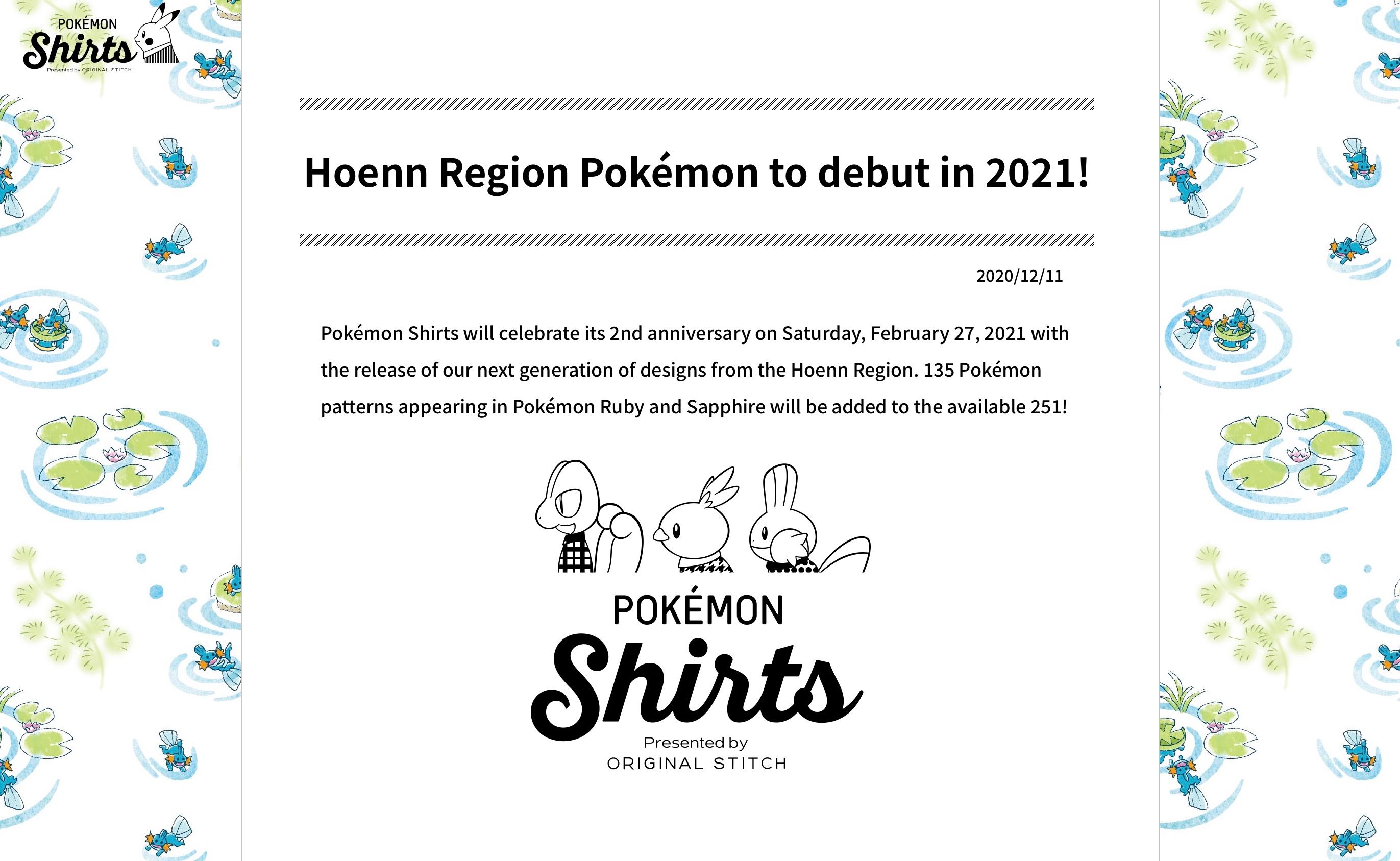The image features a vibrant, intricate design with a white border on both the left and right sides. This border evokes the tranquility of a pond, complete with green lily pads and delicate pink flowers at their centers, accented by wavy blue lines representing water. Scattered throughout are various bluish fish adorned with striking orange fins, adding a dynamic element to the scene.

At the top left corner of the image, bold black text reads "Pokemon Shirts" alongside a black-and-white illustration of Pikachu, who is gazing intently at the text. Below this, the image is divided by diagonal lines that form a subtle yet distinctive border, creating two main sections.

The central section announces: "HOENN region Pokemon to debut in 2021," presenting this information crisply between the two sets of diagonal lines. On the right-hand side, the date "2020/12/11" is prominently displayed.

Further down, in black text, the image declares an exciting update: "Pokemon shirts will celebrate its second anniversary on Saturday, February 27th, 2021 with the release of our next generation of designs for the Hoenn region. 135 Pokemon patterns appearing in Pokemon Ruby and Sapphire will be added to the available 251!"

At the bottom of the image are three distinct Pokemon characters—a fish, a bird, and a lizard-like creature—showcased against the backdrop. Finally, the caption "Pokemon Shirts presented by Original Stitch" is written in black, completing the detailed announcement.